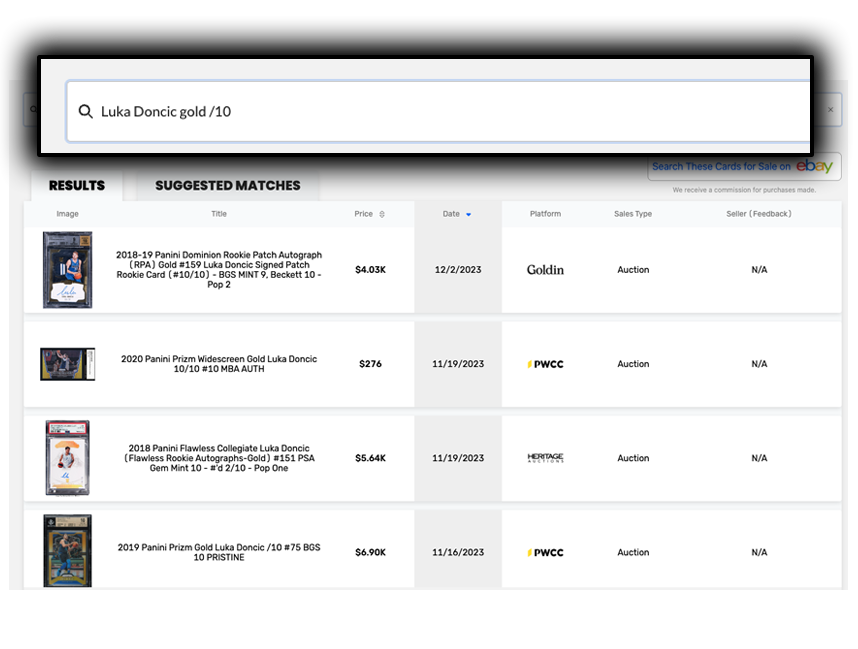On a white background, the image showcases a search interface. Positioned on the left of this interface is a magnifying glass icon next to a search bar. The results section below the search bar includes columns for Image, Title, Price, Date, Platform, Sales Type, Seller, and Feedback (noted in parenthesis).

Under the 'Image' column, there is a picture of a man playing basketball while wearing a blue jersey. The corresponding 'Title' column reads: "2018-19 Panini Dominion Rookie Patch Autograph (RPA) Gold #159 Luka Dončić Rookie Patch Card /10 BGS Mint 9 Beckett 10 Pop 2". This title signifies a 2018-2019 Panini Dominion rookie card of Luka Dončić, featuring an autograph and a patch, in gold, numbered to 10. Additional details indicate the card has been graded Mint 9 by BGS (Beckett Grading Services) with a Beckett autograph grade of 10, and a population of 2 for this grade.